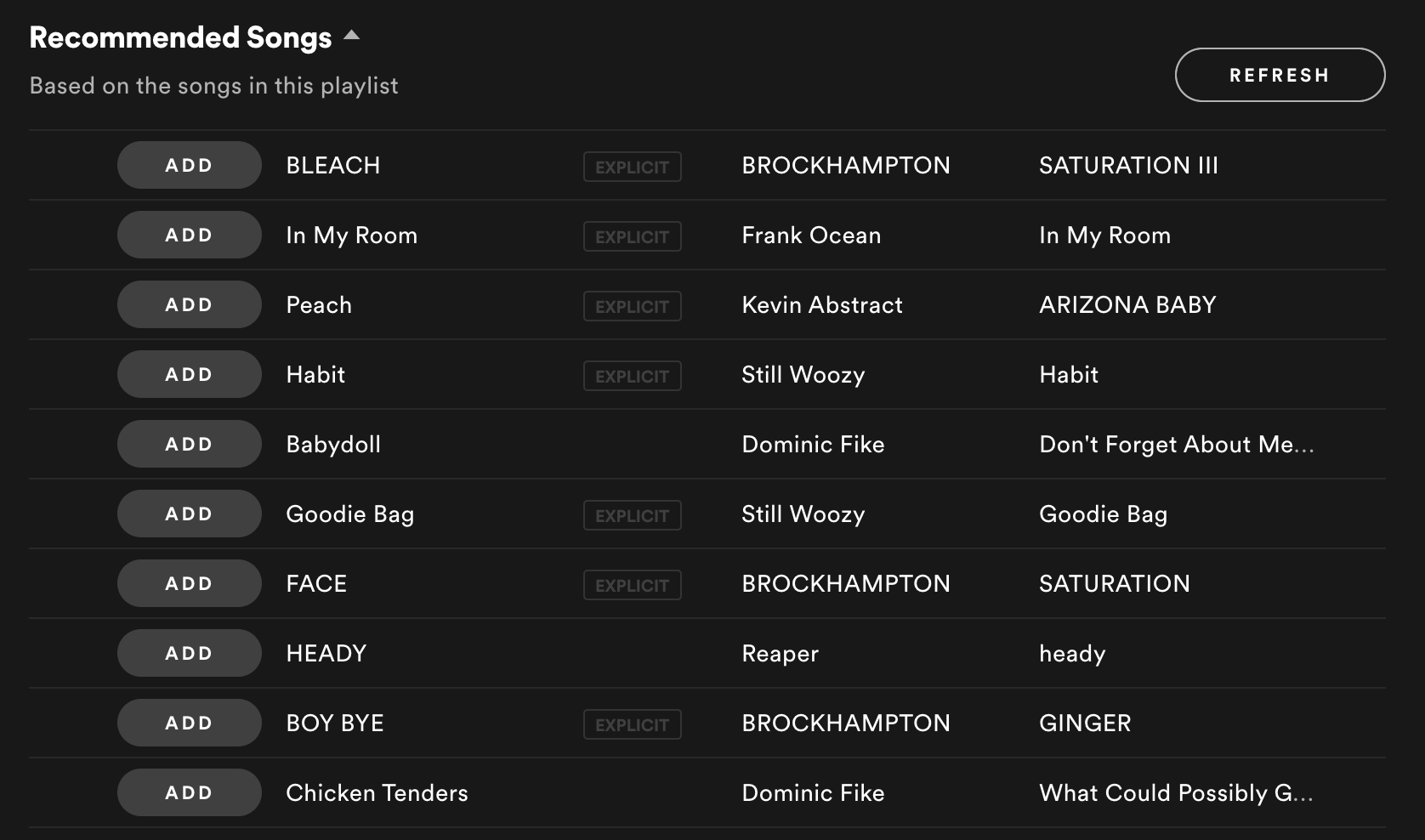In this particular photograph, we see a dark, black screen displaying a selection of recommended songs based on the contents of a playlist. The screen's interface features white text for easy readability against the dark background, providing a clean and modern look. Each recommended song has a button labeled "Add" next to it, designed in a dark charcoal gray, offering a subtle contrast to the black background while remaining distinct.

Highlighted in light white text at the top of the screen is the heading: "Recommended Songs Based on the Songs in This Playlist," indicating the nature of the selections.

Below this heading, twelve recommended songs are listed:

1. "Bleach" by Brockhampton from their album "Saturation"
2. "In My Room" [Explicit] by Frank Ocean
3. "Peach" [Explicit] by Kevin Abstract
4. "There's Not a Baby" by Have It [Explicit], performed by Still Woozy
5. "Baby Doll" by Nomadic
6. "Fight" [Explicit] by Don't Forget About Me
7. "Goody Bag" [Explicit] by Still Woozy
8. "Face" [Explicit] by Brockhampton from their album "Saturation"
9. "Petty" by Creeper
10. "Boy Bye" [Explicit] by Brockhampton from their album "Ginger"
11. "Chick Tenders" by Dominic Fike from his album "What Could Possibly Go Wrong"

Each of these recommendations is thoughtfully curated to align with the listener’s musical preferences based on the current playlist. The sleek design and intuitive layout make for a visually appealing and user-friendly browsing experience.